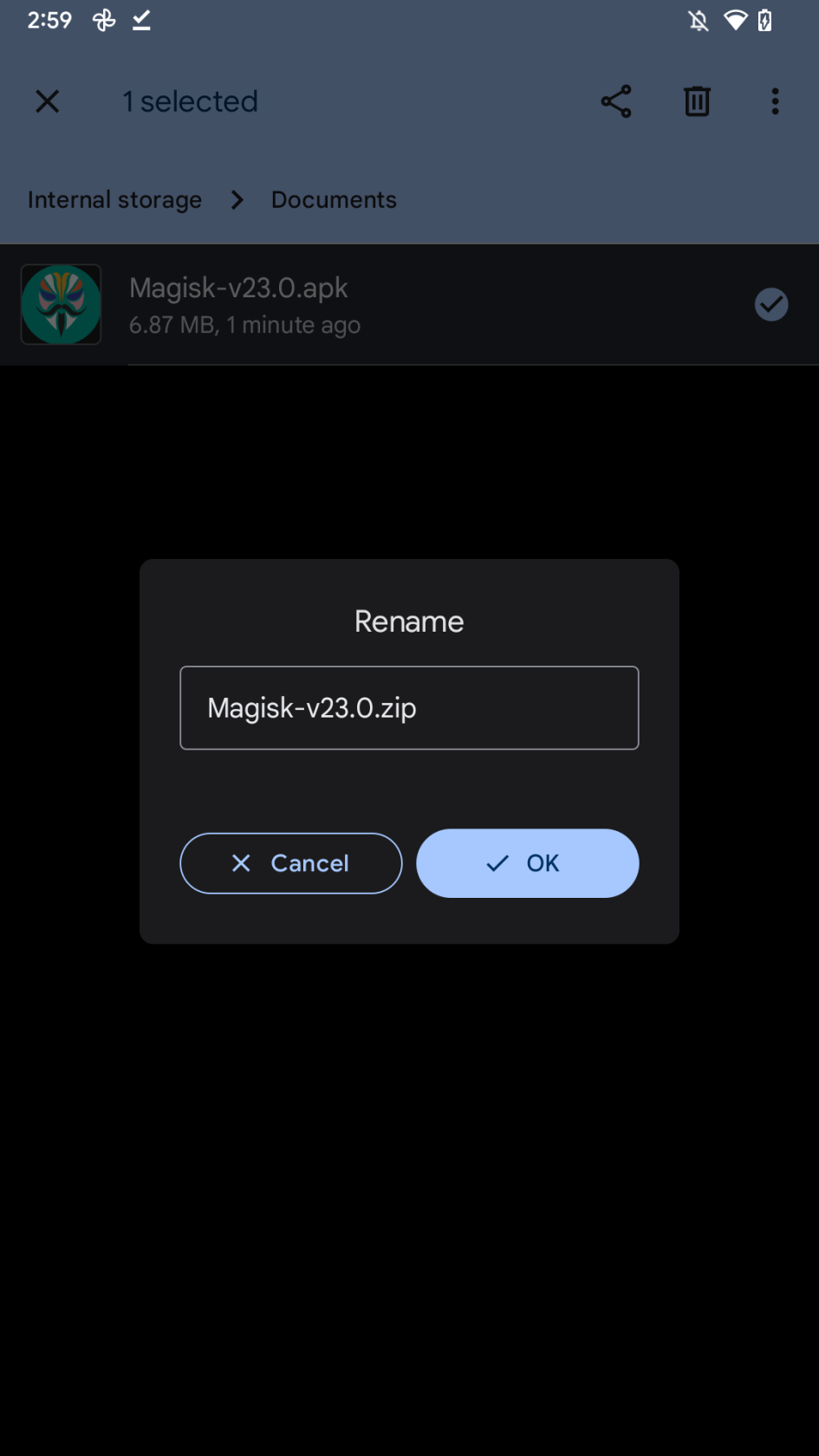The image captures a smartphone screen displaying various elements. At the very top, the time is shown as 2:59, with the battery indicator visible and notifications turned off. Below the status bar is a heading labeled "Internal Storage - Documents." 

Underneath, a gray panel spans across the screen, listing an application labeled "Magisk v23.0.apk" which is 6.87 megabytes in size and was downloaded one minute ago. To the right of this name, there is a blue tick mark and an icon resembling a mysterious figure with a long mustache and beard, colorful face—reminiscent of a magician.

Centered on the screen is a gray dialog box titled "Rename," containing an editable field with the text "magisk-v23.0.zip." Below this field are two buttons: "Cancel" and "OK," with the "OK" button highlighted in blue. The rest of the screen has a black background, providing contrast to the displayed elements.